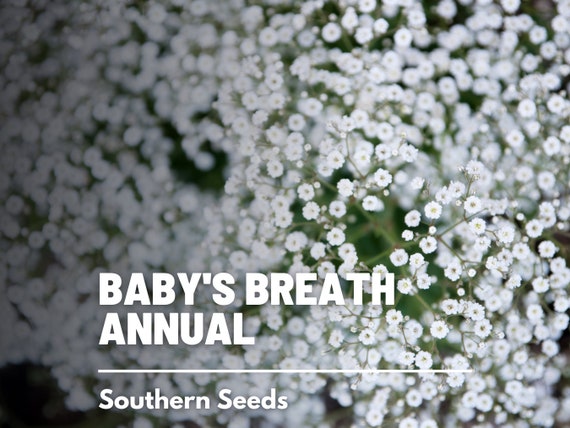This social media graphic features an extremely close-up, detailed image of Baby's Breath flowers from Southern Seeds. The composition highlights the delicate white petals and tiny yellow centers of the flowers. The part of the image that is sharply in focus showcases the fine textures and thin green stems of the Baby's Breath, while the surrounding areas blur out, creating a distinctive depth-of-field effect. The background has a greenish hue, enhancing the natural, garden-like setting. In bold white letters at the bottom, the text reads "Baby's Breath Annual by Southern Seeds," making it clear this is likely packaging for seeds. A subtle dark vignette on the left side of the graphic casts a shadow that makes the bright and intricate details on the right side stand out even more, drawing the viewer’s eye to the beauty of the finely detailed flowers.